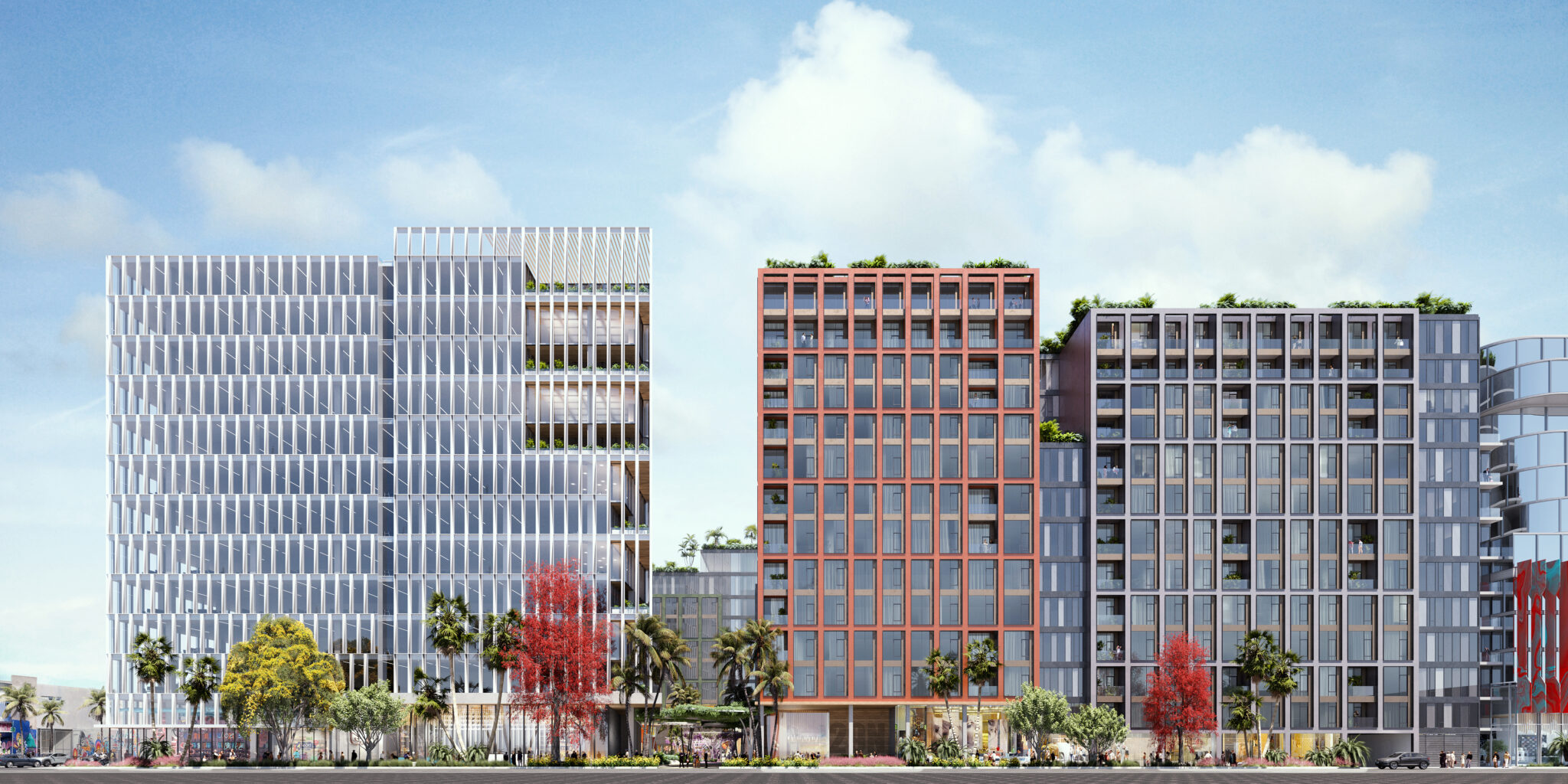The image appears to be a computer-generated or artist-drawn depiction of an urban landscape featuring three high-rise buildings, each distinct in color and design. The building on the left is white and slightly whiter than the other two. In the center, there is a narrower red building, and to the right, there is a silver building of moderate width. All three buildings are approximately six stories high and are characterized by large, glass-paneled facades. 

In front of these buildings, a variety of trees are visible, including numerous palm trees, smaller green trees, and two distinct trees with red leaves and grey trunks, suggesting a fall season. The background features a partially cloudy blue sky. Additionally, multiple people can be seen milling about in the foreground, giving the scene a populated and lively atmosphere. There are also bushes and occasional vehicles, such as an SUV on the right and other cars dispersed on the left side, completing the cityscape.